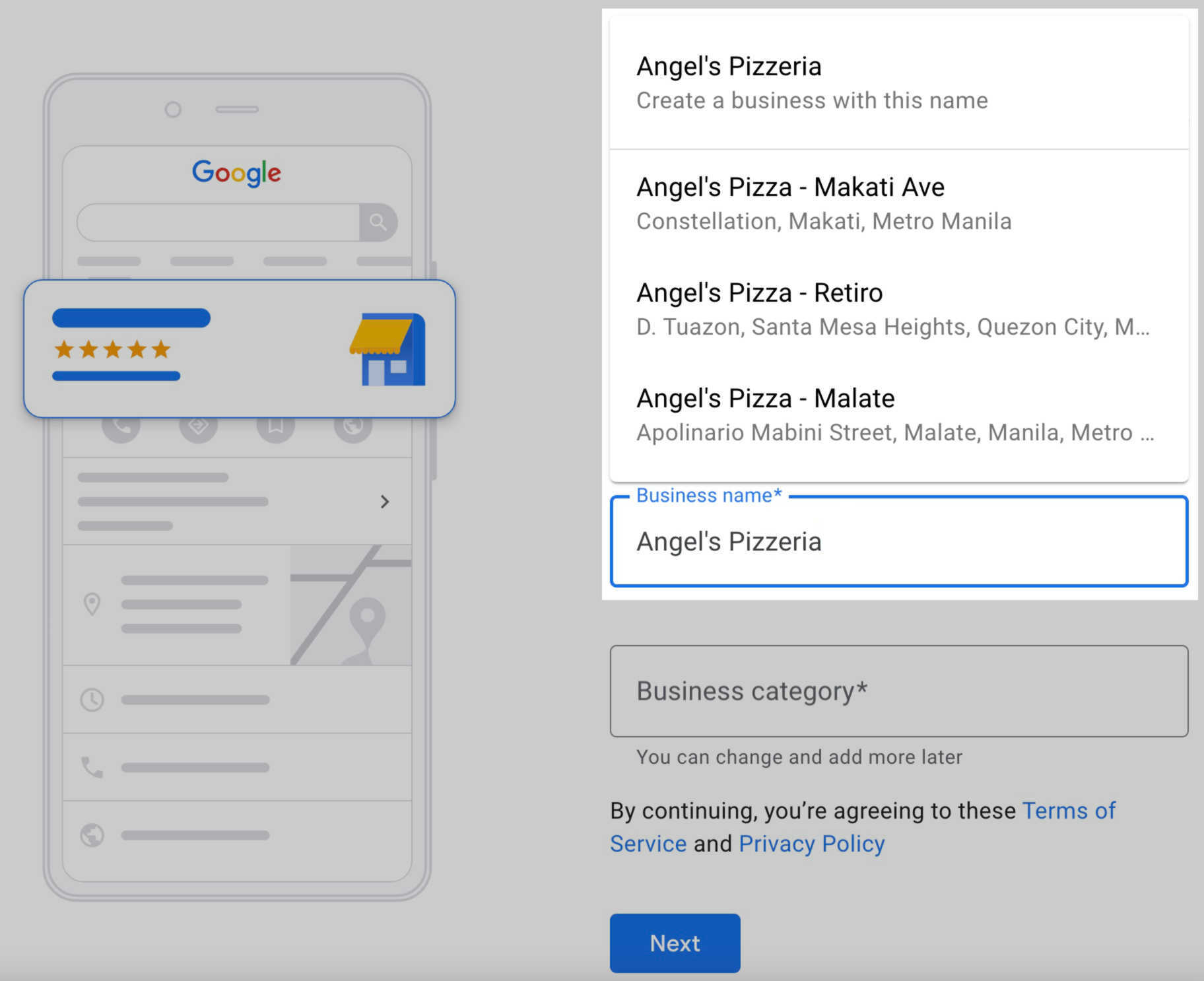The screen displays a web page from Google My Business, showcasing an interface for searching and rating businesses. On the left side of the page, there's a prominent graphic featuring the Google logo alongside icons representing business searches and a five-star rating system, highlighting the functionality for users to leave reviews and rate businesses. The user seems to be searching for "Angel's Pizzeria," as indicated under the business name search field. A dropdown menu presents several possible matches: "Angel's Pizzeria," "Angel's Pizza, Makati Avenue," "Angel's Pizza Retiro," and "Angel's Pizza Malate," offering different locations of the same or similarly named establishments. Additionally, there is a section where users can list the business category. The image captures the detailed interaction with Google My Business, aimed at managing or locating specific business listings.